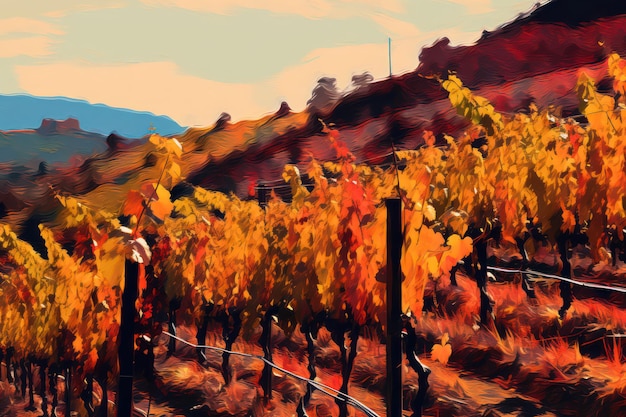This painting depicts a vibrant vineyard sprawling across a gently undulating field. Three distinct rows of grapevines, supported by wire-fenced structures, stretch horizontally across the scene. The grapevines, adorned with leaves that have turned a fiery palette of amber, yellow, and orange, juxtapose against the lush green rows of grass at the base. In the background, a series of rolling hills create a gradient of hues - from the light, muted blue of the furthest hills to the rich, amber and red tints of the closer ones. These hills, along with the scattered clumps of vegetation, add depth and dimension to the landscape. Dominating the distant horizon is a prominent blue hill, shadowed against the cloudy, white sky that gradually transitions into a clear blue as it climbs higher. The painting skillfully captures the intricate details of the grapevines up close, while the background elements, including a solitary pole and indistinct trees, blur softly into the distance, embodying the essence of a serene vineyard amid autumn's embrace.